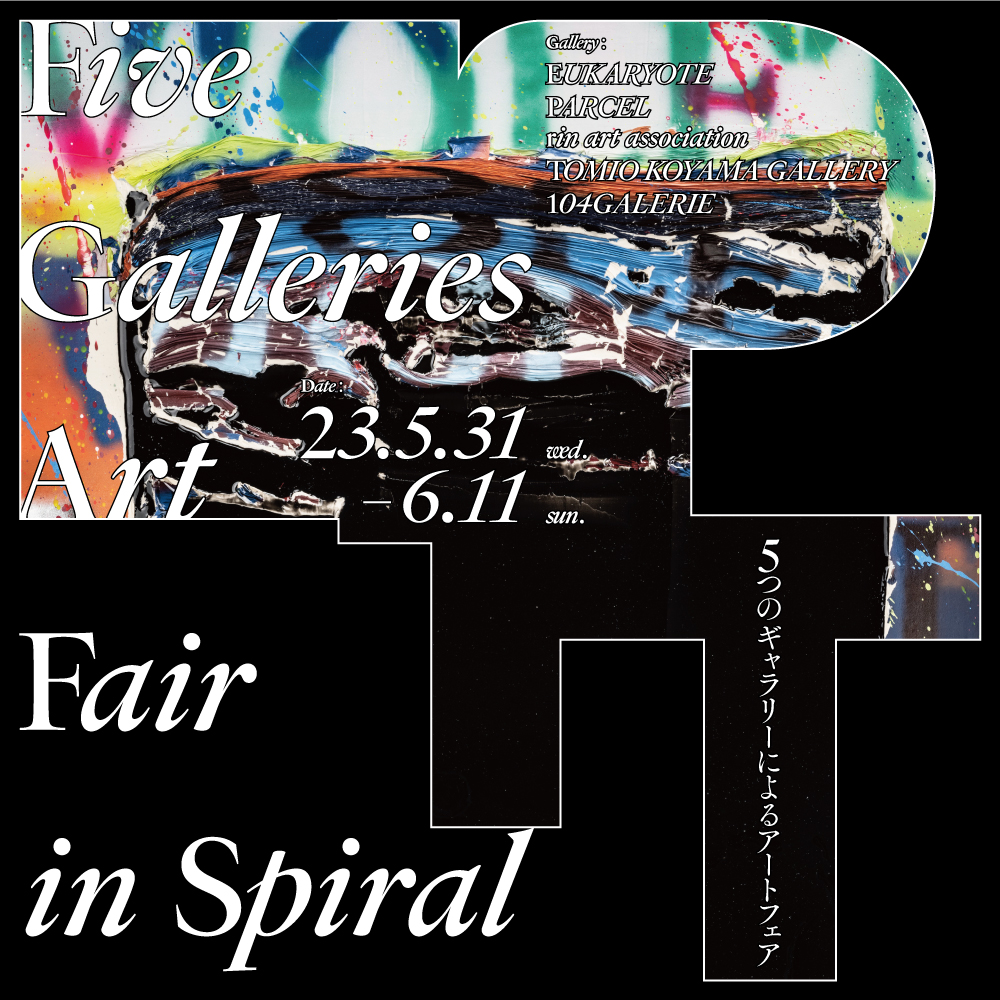This poster advertises an art gallery event in Japan, set against a solid black background. It prominently features an abstract collage of swirling colors—including blues, whites, blacks, oranges, pinks, yellows, greens, and creamy whites—evoking the appearance of flowing water and dramatic brushstrokes. Central to this poster is a puzzle piece-like shape outlined in white, containing various fragments of information and artwork. 

The centerpiece text in bold white letters reads "5 Galleries Art Fair in Spiral," with the event dates "23.5.31 Wednesday through 6.11 Sunday." Additional text within the puzzle piece lists the participating galleries: "Eukaryote, Parcel, Rin Art Association, Tomio Koyama Gallery, and 104 Gallery." There is also a vertical line of non-English text, likely Japanese, providing further details or an address. Inside the puzzle piece, there's an abstract painting with splashes of blue, black, and mauve. The entire composition combines textual and visual elements to create a vivid and dynamic advertisement for the upcoming art fair.